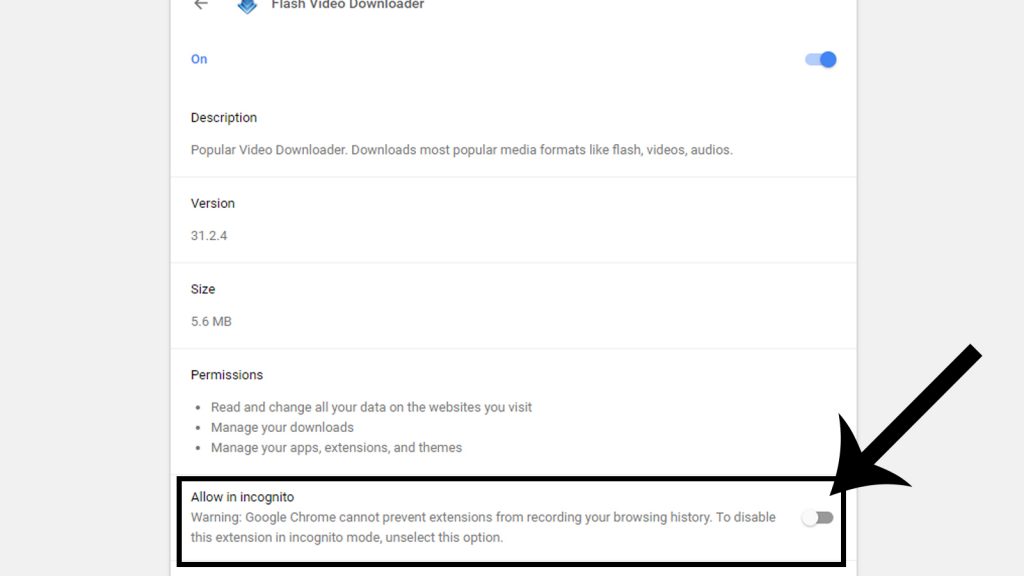The image is a screenshot of a software interface titled "Flash Video Downloader". At the top, the title "Flash Video Downloader" is prominently displayed. Below this, a toggle button labeled "On" is turned on, indicating that the downloader is currently active.

The next section provides a detailed description of the software, listing its capabilities: "Popular video downloader downloads most popular media formats like flash videos and audios." This is followed by version information: "Version 31.2.4," and the download size: "5.6 MB."

Permissions required by the software are listed as follows:
- "Read and change all your data on the websites you visit."
- "Manage your downloads."
- "Manage your apps, extensions, and themes."

At the bottom of the screenshot, there is a highlighted section enclosed in a bold black rectangle, emphasizing the option "Allow in Incognito." Alongside this, a warning reads: "Google Chrome cannot prevent extensions from recording your browsing history. To disable this extension in incognito mode, unselect this option." To the right of this text, there is a toggle button which is set to off, indicating that the extension is not allowed in incognito mode. Additionally, this section features a bold black arrow pointing towards the box, with no arrow pointing down into it.